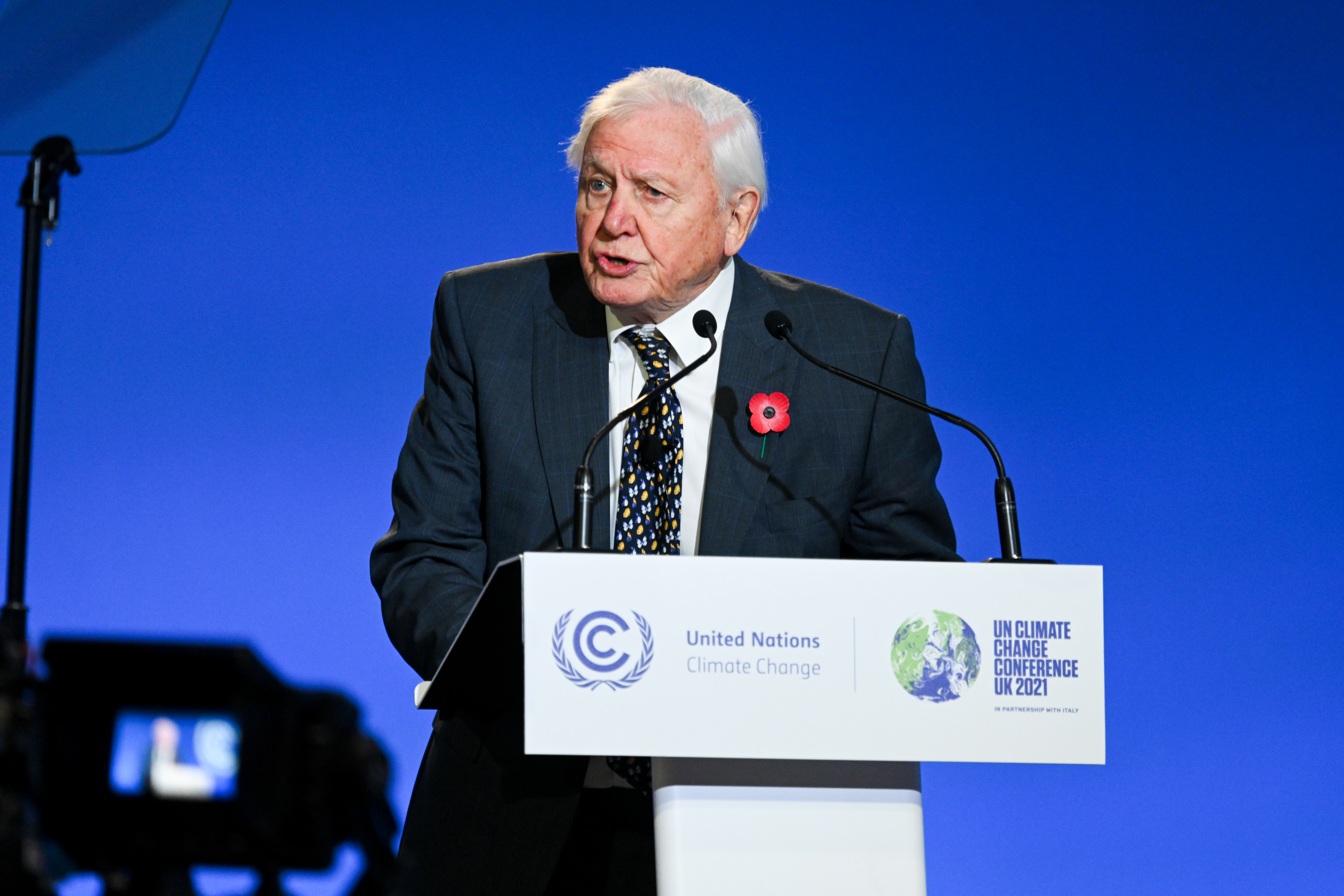This image captures an elderly white man, likely in his 60s or 70s, with medium-length grey to silver hair, and age spots, standing indoors at a podium. He is mid-speech, looking slightly away from the camera, and the setting appears to be a convention or meeting. The man is dressed in a grey suit adorned with a poppy on his lapel, a white collared shirt, and a black tie with yellow and blue accents. 

The podium, predominantly white, features a graphic with the letter "C" entwined with laurel leaves, representing the United Nations Climate Change. The text "UN Climate Change Conference UK 2021" is also displayed, suggesting the event took place in partnership with Italy, though the smaller text isn't fully readable. Behind the man, a vivid blue background contrasts with a television screen showing a smaller, blurrier image of him. Two microphones are affixed to the podium, along with an additional screen located in the top left corner of the image.